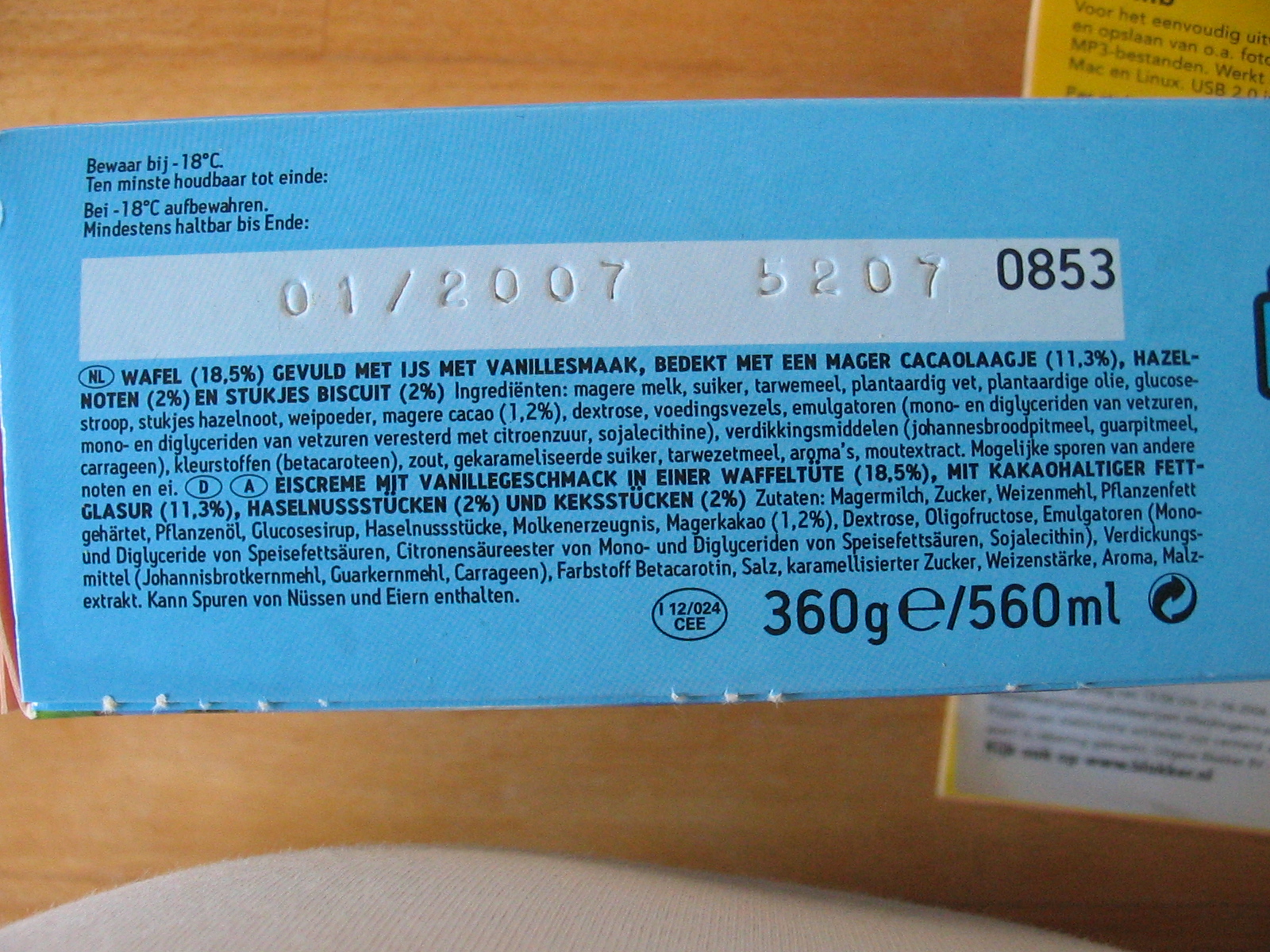The image displays a portion of a food package in landscape orientation. The packaging is primarily blue, composed of what appears to be a cardboard material. Dominating the upper part of this section is a narrow, white rectangular shape, embossed with a series of numbers "01-2007," followed by a space and another series "5-2-0-7." Below these embossed numbers, there is a string of black-text digits reading "0-8-5-3." Underneath this numeric information, the package features a typical list of ingredients, printed in a language that resembles German. The ingredients list is also laid out within this narrow, rectangular section, contributing to the overall detailed information present on the small area of the packaging being observed.